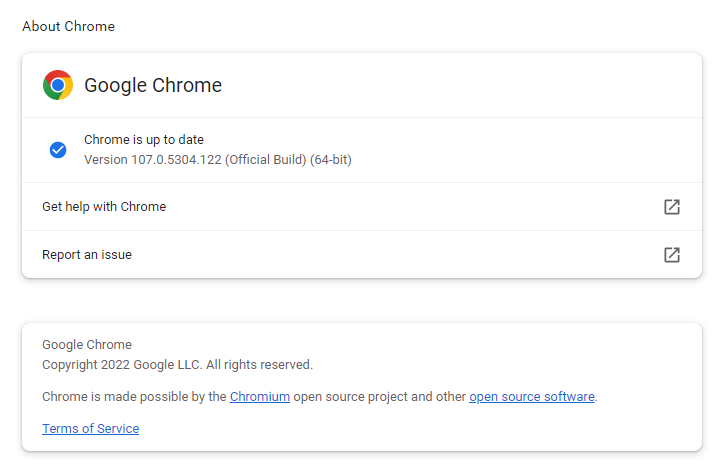The image showcases the Google Chrome browser interface in detail. On the left, the iconic Google Chrome logo is prominently displayed, featuring a circular design with sections of red, yellow, and green surrounding a blue center. To the right of the logo, the text "Google Chrome" is clearly visible.

Beneath this header, a thin gray line separates the sections of the interface. The first row includes a blue check mark and the text: "Chrome is up to date, version 107.0.5304.122 (Official Build) (64-bit)." Another thin gray line divides this from the next row.

The following section is labeled "Get help with Chrome," accompanied by an arrow inside a box icon pointing up and to the right on the far right side. Another thin gray line leads to the next row, which reads "Report an issue," also paired with a similar gray arrow box icon.

At the bottom of the image, a distinct gray rectangular area states: "Google Chrome, copyright 2022, Google LLC, all rights reserved. Chrome is made possible by the Chromium Open Source Project and other open source software." Hyperlinks are provided for "Chromium Open Source Software" and "Terms of Service."